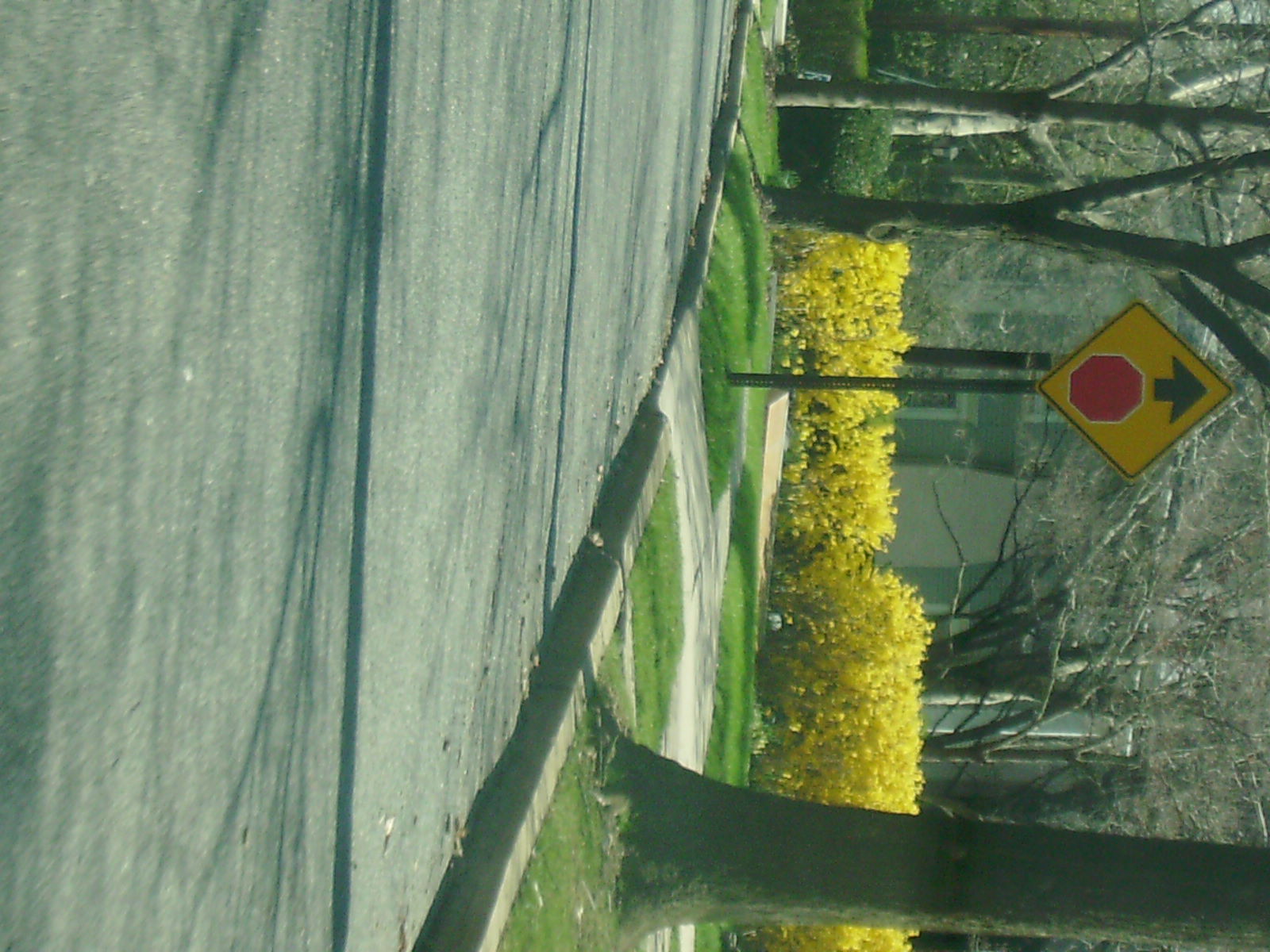A peaceful street scene on a sunny day, captured with the photo turned a quarter to the right. The image reveals a quiet road flanked by a row of verdant trees standing on lush green grass. Beside the trees runs a cement sidewalk, beyond which lies more green grass followed by a line of yellow-flowered bushes. Along the sidewalk, a metal pole holds a yellow diamond-shaped sign featuring an image of a red stop sign outlined in white with a black arrow above it, indicating an upcoming stop sign. In the background, behind the vibrant bushes, stand leafless trees and a stately stone building. The building, with its gray stone facade, features sections of green paint and a white-painted door entryway.